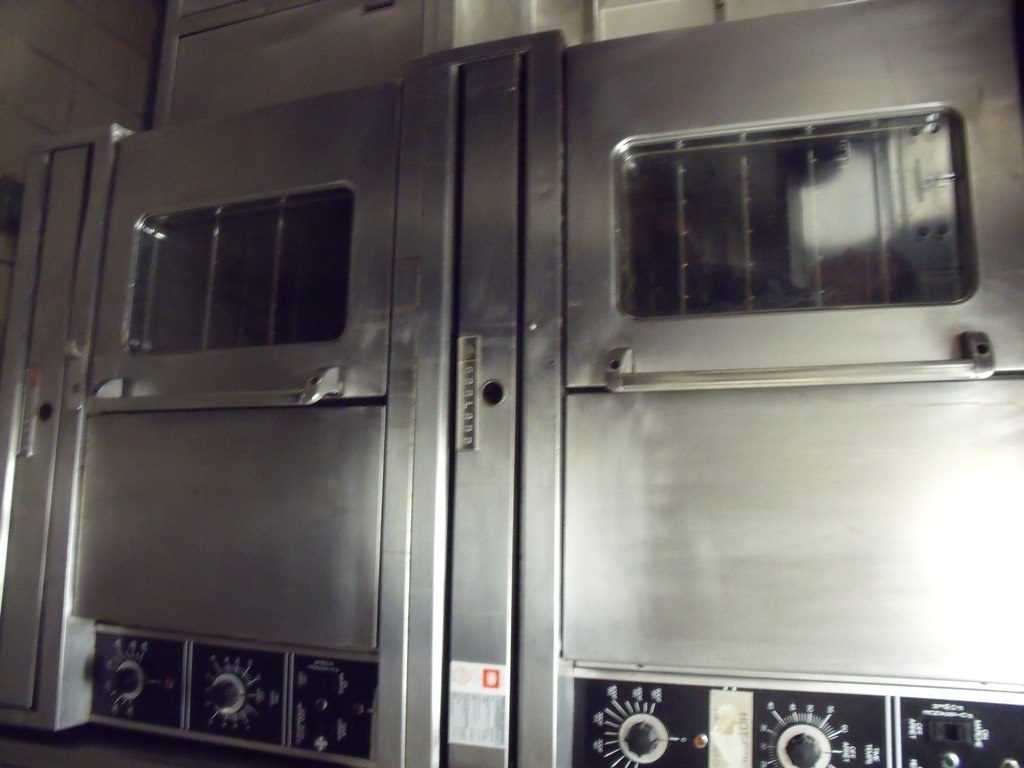This close-up photograph features two large, identical pieces of stainless steel machinery, which are most likely kitchen ovens, although they could be mistaken for scientific equipment. Dominating the image, these ovens exhibit a polished silver chrome finish. Each oven has a prominent rectangular door at the top, featuring a smaller inset window made of glass, reinforced with metal bars, for viewing the interior wire racks. These doors are equipped with large, silver handles for easy operation. Below the glass window on each unit, there's a panel consisting of three sections with a black background. The left section contains a switch, while the other two sections are fitted with dials marked with numbers and white labels, presumably for controlling temperature or other settings. The background showcases a white wall lined with rectangular tiles, providing a clean and sterile environment.